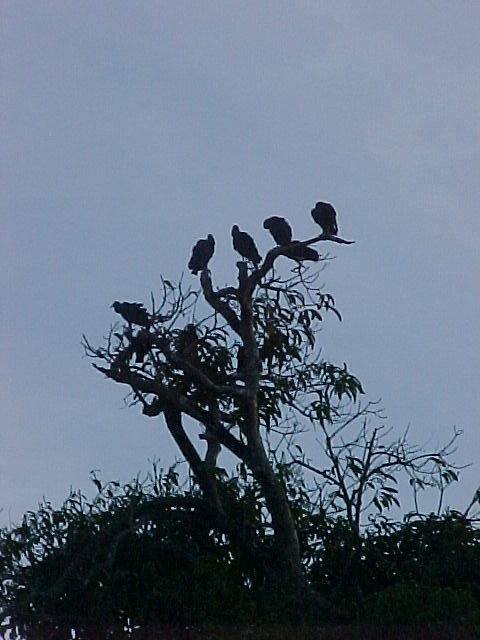This photograph, possibly taken after sunset due to the poor lighting, captures the silhouette of a barren treetop against a dark, uniform grey-blue sky. The image centers on the upper part of the tree, where several large birds, their details obscured in the silhouette, are perched. There appear to be at least six birds, with four occupying the topmost branches and two situated slightly off to the left. The branches, stark against the dim sky, show not only the primary limbs but also smaller twigs and minimal foliage below, where you can discern the outlines of additional bushes or shorter trees. Despite the blurriness of the photograph, the stark contrast between the dark tree and birds against the grey backdrop creates a distinct and evocative image.